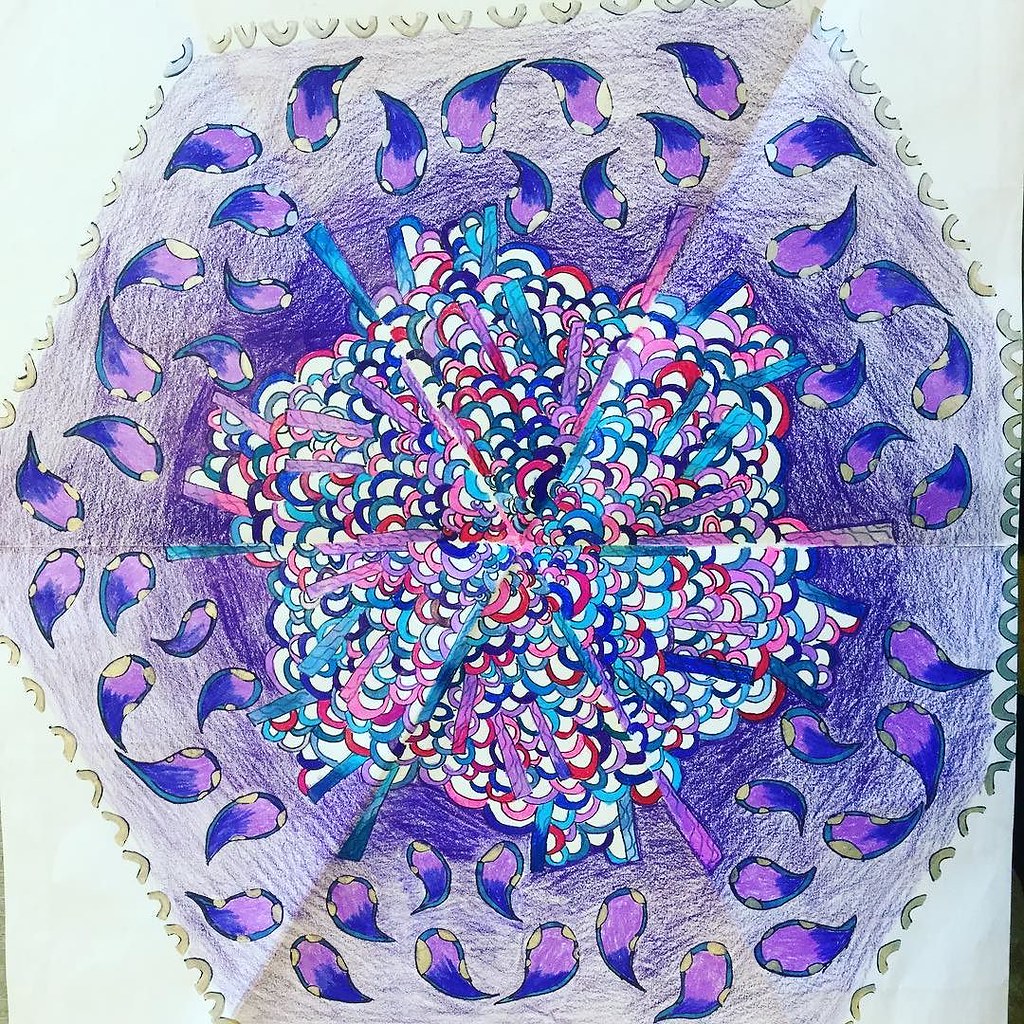This is an illustration meticulously crafted with colored pencils and markers, set against a white background. The drawing depicts an intricate seven-sided shape, bordered by evenly spaced, silver-colored upside-down U's. Inside this heptagon, the central focus is a starburst pattern composed of concentric half-circles in varying hues—white centers outlined with dark blue, light blue, red, pink, and purple. Surrounding this central motif are teardrop-shaped elements in shades of dark purple and light purple, accented with blue borders and white spots. The outer edges feature curved, light green designs, creating a harmonious frame. Adding further detail, there are scattered, raindrop-shaped droplets colored purple and blue, resembling petals dispersed throughout the composition. These elements combined evoke the intricate beauty of a mandala infused with vibrant colors and delicate shading.